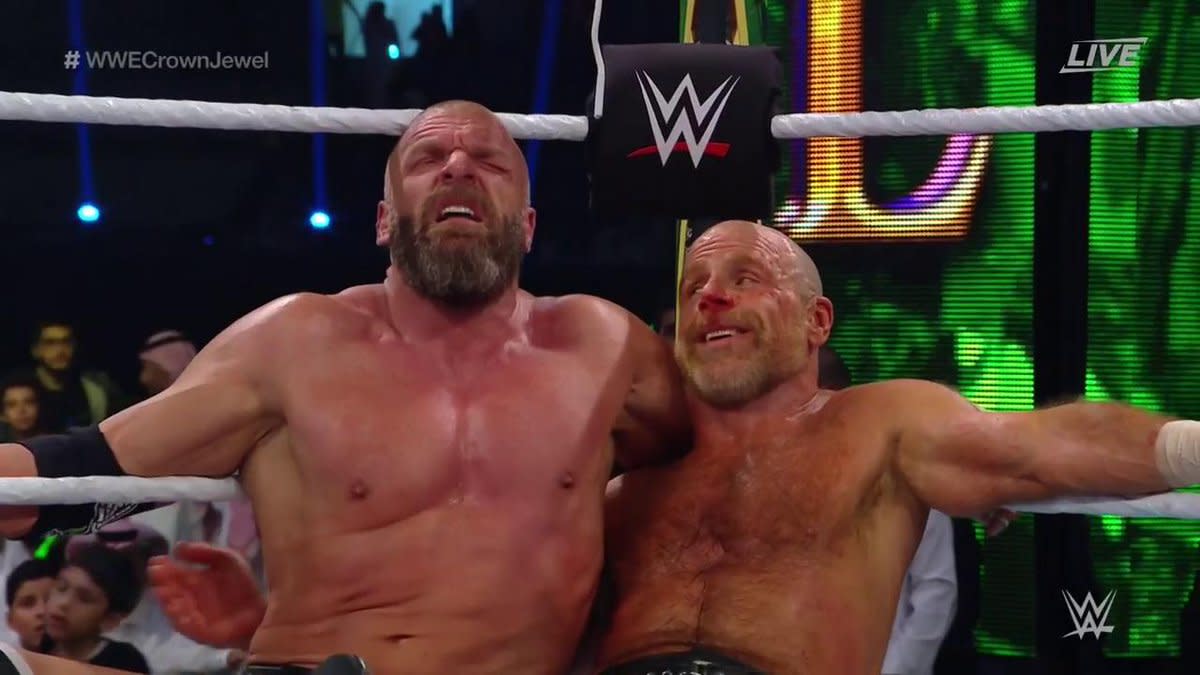In an intense wrestling match, two shirtless wrestlers are leaning against the white ropes in a corner of the ring, both appearing exhausted and in pain. The wrestler on the right has a light blonde beard, a mostly shaven head, a hairy chest, and a bloody nose. His right arm clutches the ropes for support. The wrestler on the left, noticeably more muscular and hairless on his chest, sports a dark black beard and squints his eyes closed as he hooks his arm around the ropes. Overhead, a black square displays the WWE logo in white with a red underline, and "Live" is written in gray in the upper right corner. "Hashtag WWE, Crown Jewel" is prominently featured in the top left corner. The bottom right corner also showcases another WWE symbol. The background captures the excitement of the venue with green fluorescent lights on the right and glimpses of the audience on the left, emphasizing the indoor setting and bustling atmosphere. Subtle details in the scene include a random hand emerging from the bottom left, possibly belonging to an unseen participant or an audience member nearby.